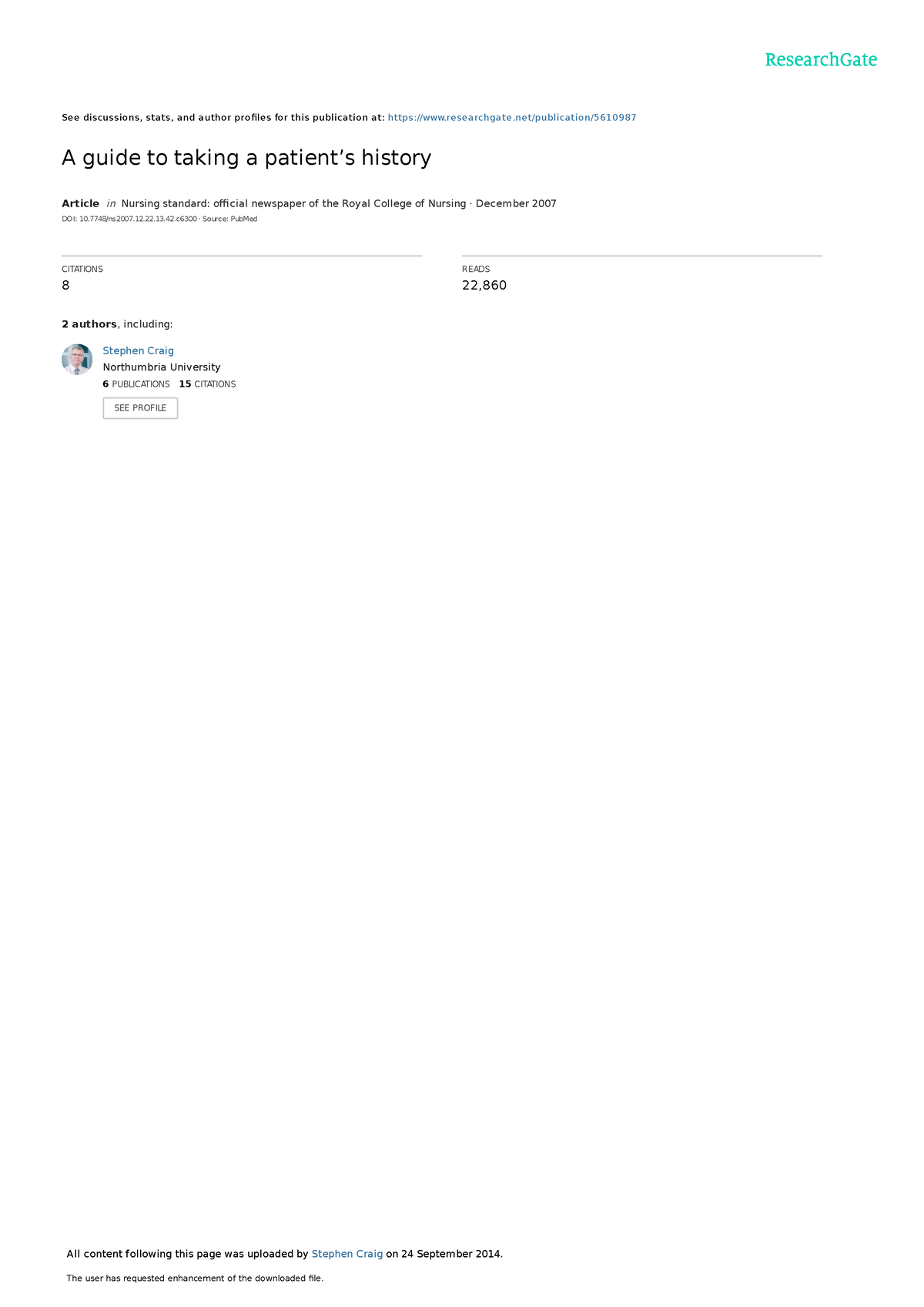This image displays a webpage from ResearchGate, dedicated to a guide on taking a patient's history, likely targeted at healthcare professionals such as doctors and nurses. The website's name, "ResearchGate," is discreetly placed in small green text on the right-hand side, which could benefit from being more prominent for better visibility. The main title, "A Guide to Taking a Patient's History," is intended to support medical staff in triage procedures by offering various methods for efficient patient history documentation.

The page contains an article section, marked by the word "Article" in black text, which provides a brief overview of its contents. Accompanying this article are eight comments situated below the main text. On the right-hand side of the webpage, there is a small image of a man, presumably Steven Gregg, associated with a university. He appears to be dressed formally in a suit and tie, suggesting he may be a respected professional or contributor to the article. Beside his image is a numeral, "22,860," which could indicate the number of views, downloads, or citations related to his work.

Overall, the page lacks a professional and engaging design, as it features a plain white background with minimal visual elements. The lack of color and imagery makes the webpage appear uninviting and bland, underscoring the need for enhanced visual appeal to create a more welcoming and polished user experience.